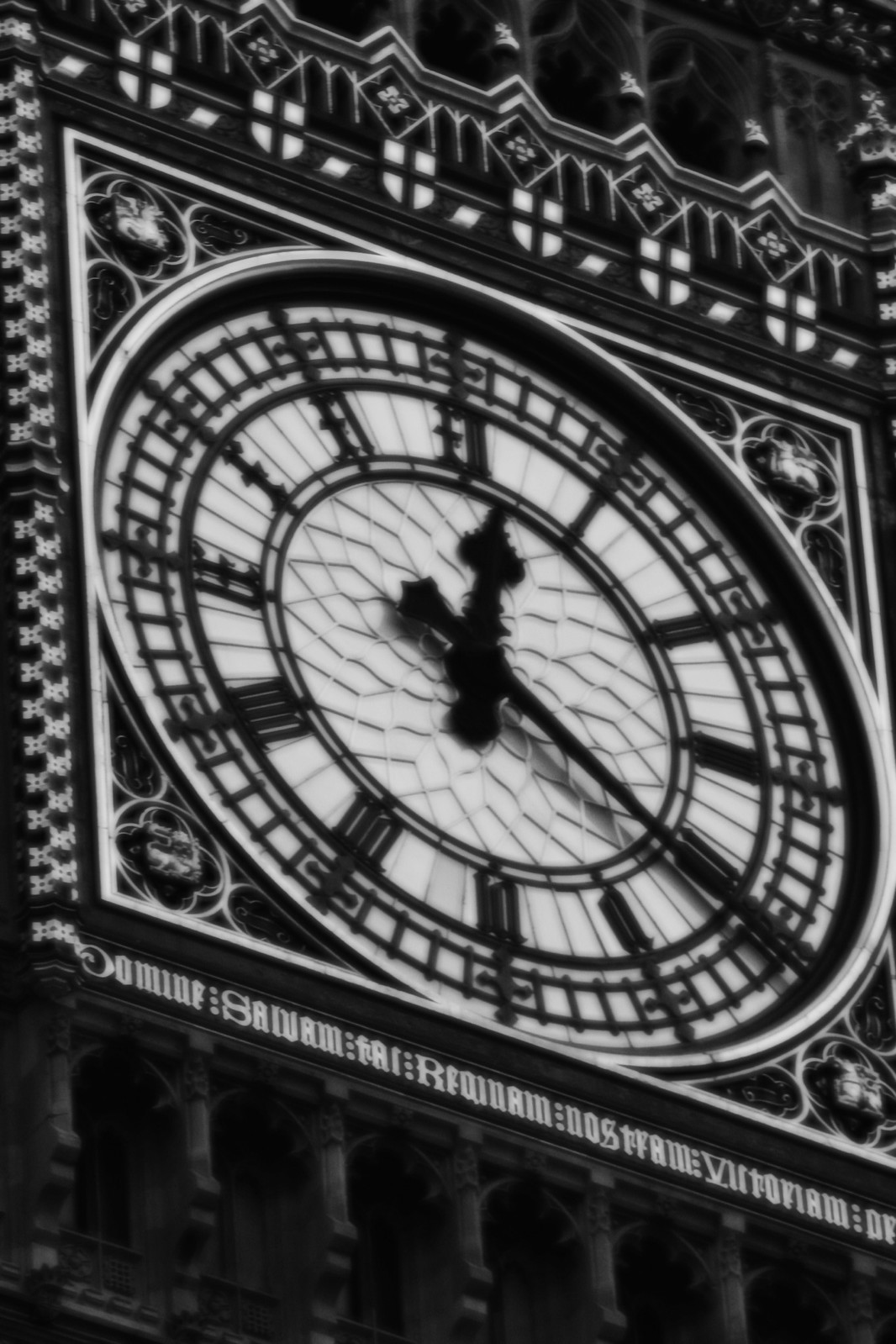This black and white image captures a close-up view of a grand, ornately designed clock situated high upon a city square tower. The clock is embedded within a square frame that encloses a circular clock face at its center. Gothic architectural details are prominently displayed, with intricate patterns and decorations crafted from what appear to be metallic wires.

The clock face itself is marked by unique symbols representing the hours, arranged in a distinctly gothic style. Its hour and minute hands point to approximately 12:20. Beneath the square frame, there is some text that seems to be in Latin, possibly containing the word "Requiem," and features Roman numerals and medieval-style lettering, further enhancing the historical ambience.

This image is a mesmerizing study of the harmony between functionality and elaborate design, perfectly capturing the timeless elegance of gothic architecture and its ornate craftsmanship.